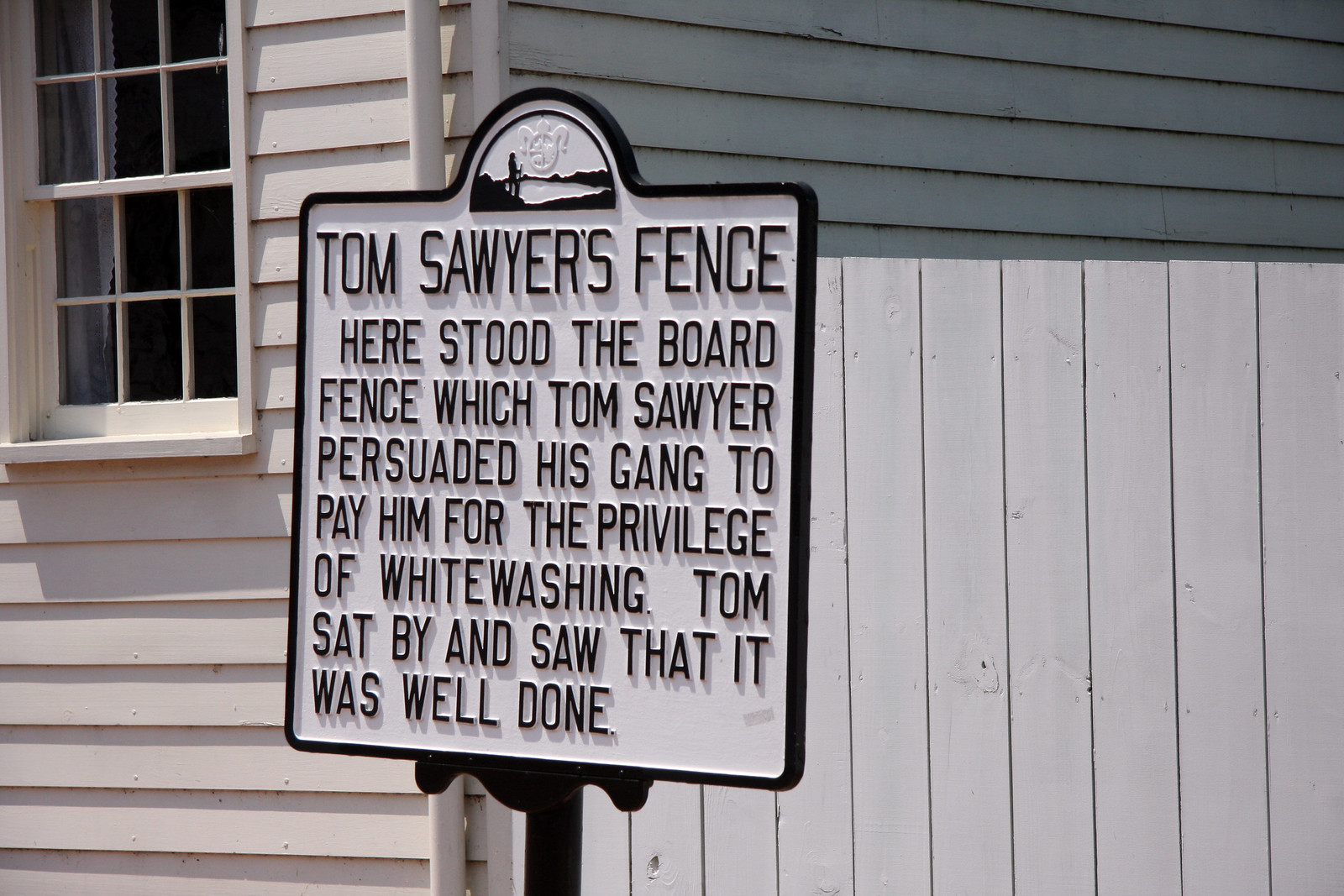In the image, there is a prominently displayed white sign with black text and a black border, mounted on a black pole. The sign reads, "Tom Sawyer's fence. Here stood the board fence which Tom Sawyer persuaded his gang to pay him for the privilege of whitewashing. Tom sat by and saw that it was well done." At the top of the sign, there is a black-and-white illustration showing someone overlooking a lake. 

Behind the sign, there is a white board fence, the subject of the text, and further back is a white building with a window, possibly a house. The surrounding details add context to the significance of the fence, highlighting its cultural and literary reference to Mark Twain's famous novel, "The Adventures of Tom Sawyer."